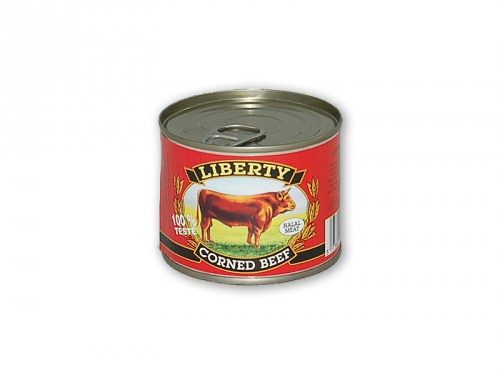This close-up image features the front of a small metal can of Liberty corned beef on a transparent background. The can has a pull tab top and is adorned with a detailed red label. Central to the label is an oval containing a picturesque scene of a cow standing in a green pasture with a blue sky backdrop, symbolizing the quality of the meat. This oval is flanked by curved wheat stems, elegantly framing the image. Above this central oval, a black banner with gold trim prominently displays the word "Liberty" in gold lettering. Below, another black banner with a gold outline bears the words "corned beef" in white writing. On the left side of the label, overlaid text reads "100% tested," while an oval on the right side indicates the product is "halal meat." A partial image of the barcode is visible on the right side. The entire composition of the label combines elements from both descriptions, emphasizing the careful detailing and quality assurances presented on the product's packaging.